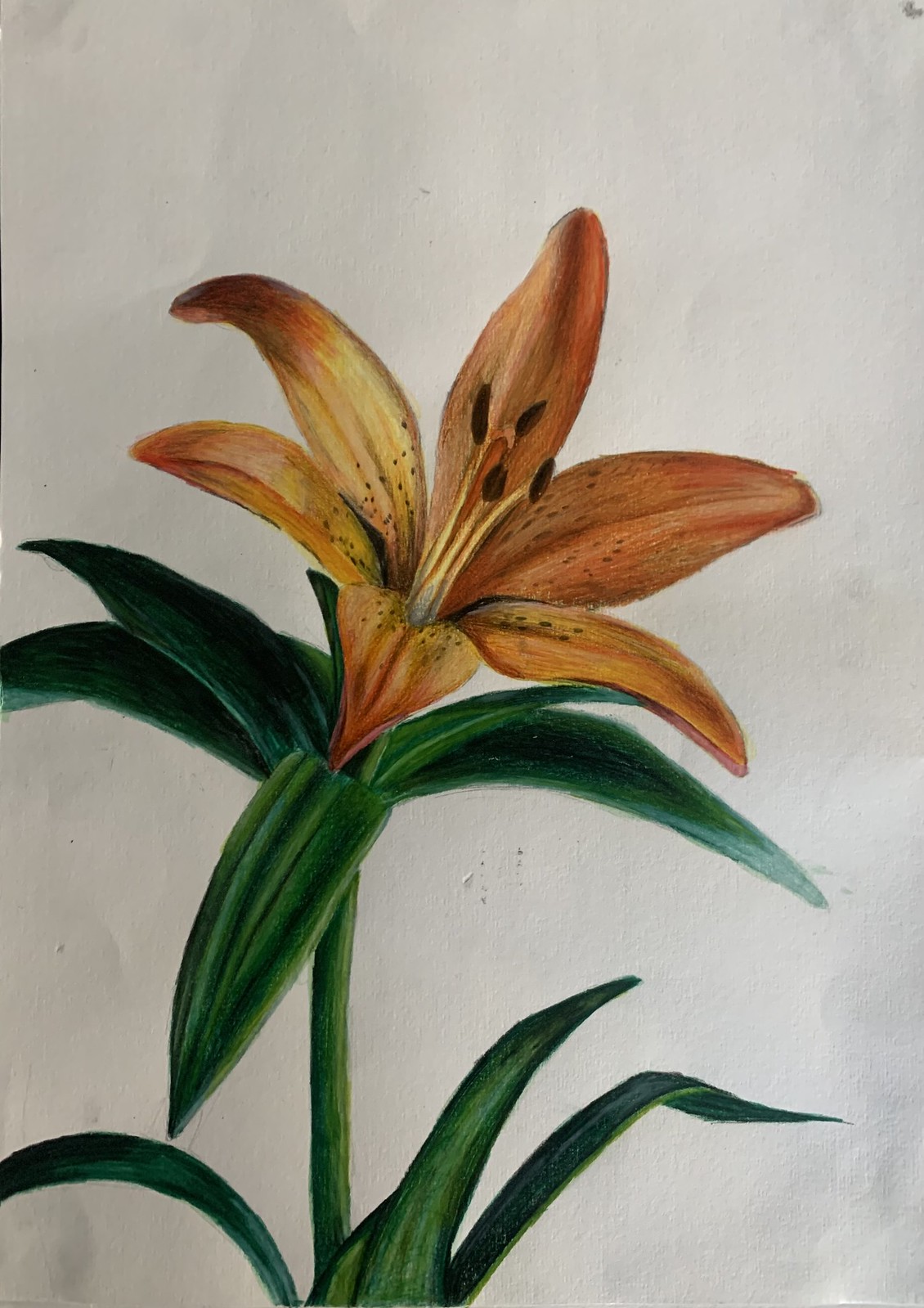This is a meticulously drawn image of a vibrant tiger lily rendered with colored pencils. The vividly orange flower is set against a plain white sketchbook background, highlighting its intricate details. The lily features a green stem that arises solo from the bottom of the page, accompanied by four blade-like leaves at its base. As the stem ascends, additional leaves emerge, curving gracefully—one in the foreground, two on the right, two on the left, and one subtly peeking from behind. The lily's bloom is divided into six petals, three standing erect at the back and three elegantly arching downward in the front. At the floral heart, four slender stamens extend outward, each tipped with a tiny brown anther, completing this exquisite botanical illustration.